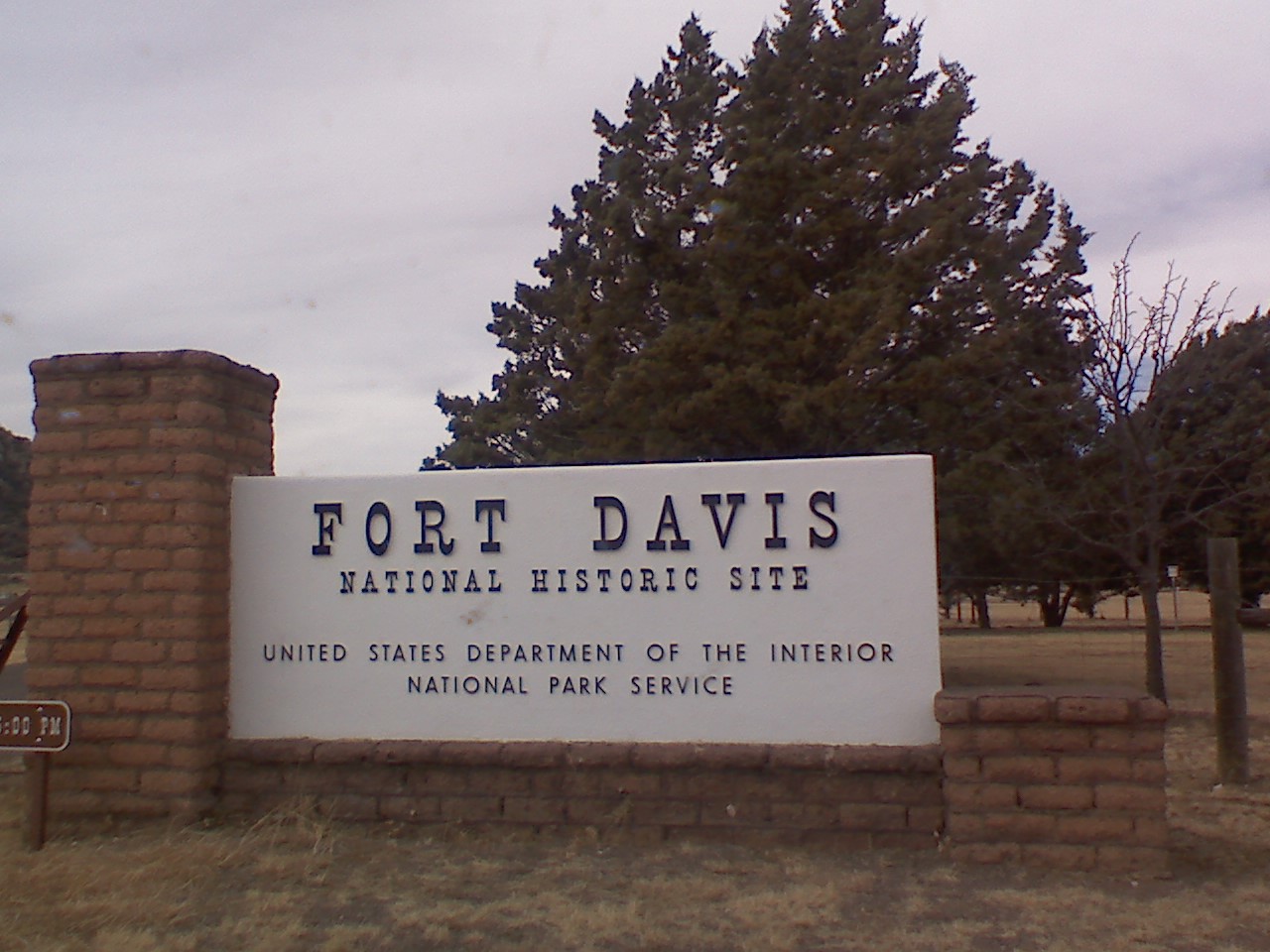The image depicts an outdoor scene centered on a historic site sign. The sign reads "Fort Davis National Historic Site" in large black lettering on a white background, with "United States Department of the Interior National Park Service" noted below it. The sign is mounted on a brick wall, which features a taller brick column on the left and a shorter one on the right. A small brown sign with partially visible hours (ending in "00 p.m.") is situated slightly to the left of the main sign. Behind the wall, there is a wooden fence with a couple of tall evergreen trees looming in the background. The photo appears to be taken on an overcast, cloudy day, hinting at fall or winter, as the grass is brown and looks dead.